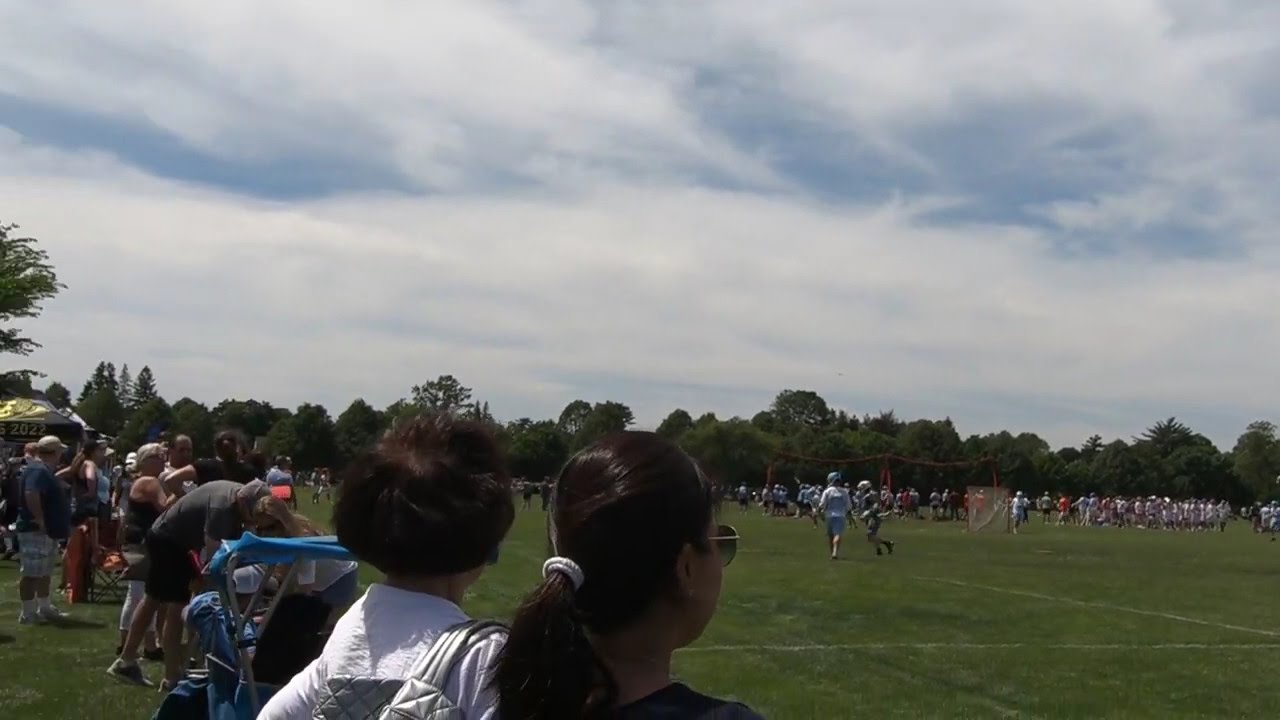The image captures a scene from what appears to be a men's lacrosse game on a hazy day at Sun Carpet Park. The field is surrounded by a scenic tree line, with the sky overhead filled with dull white clouds interspersed with hints of blue. In the foreground, several spectators are gathered along the sidelines, many with their backs turned to the camera. Prominently, there are two women: one with long, dark hair tied in a ponytail and wearing sunglasses, and another with shorter brunette hair in a white sweatshirt or coat. Nearby, a young girl stands, possibly a daughter, indicating a family presence. On the field, numerous players are actively engaged in the game, wearing protective gear typical for lacrosse. In the background, more players and spectators are visible, along with a small lacrosse goal. To the left, a concession stand serves the crowd. The overall look of the image suggests it is an older photo, with muted colors and slightly blurred details, conveying a nostalgic feel.